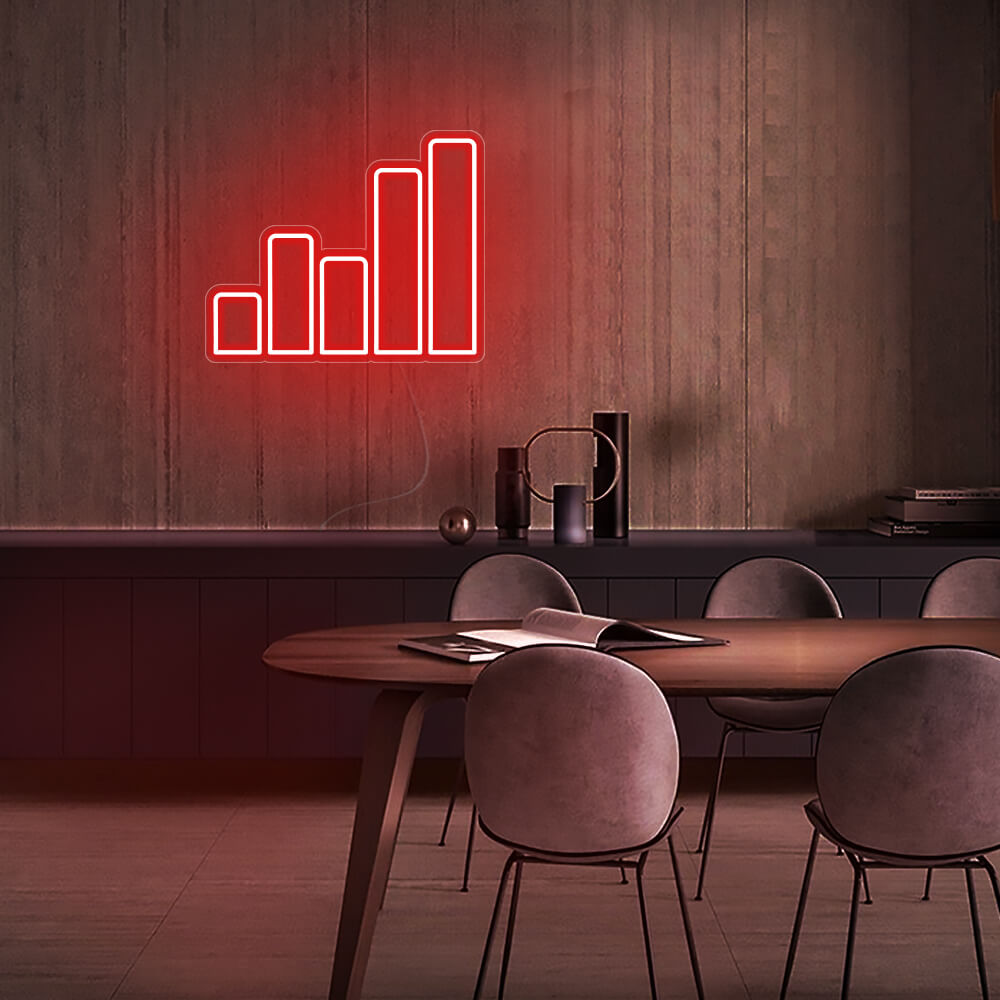This image depicts a modern conference room with a rich, brown-toned color palette. The room features an oval-shaped wooden table centrally positioned in the foreground, atop which lies an open book displaying white pages. Surrounding the table are five contemporary chairs with round backrests, brown seating, and thin metal legs. The floor is made of wood planks, maintaining the room's earthy tonal consistency. 

In the background, a wall of wood paneling extends across the length of the room, incorporating a built-in dark gray or brown counter. This counter holds an assortment of items, including a gold spherical object, three cylindrical pieces of varying colors and heights, and a stack of three books situated in the back-right corner. 

Above the counter on the wooden wall, an illuminated neon sign composed of five vertical bars of differing heights creates a silhouette that resembles a bar graph or city skyline. Each bar emits a bright reddish or orange hue, framed by white lights, contributing a modern, artistic aesthetic to the room.